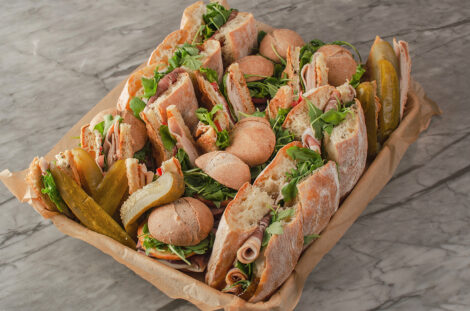This is a detailed photograph of a box full of sandwiches, resting on a gray mottled marble countertop with lines of brown, black, and some white splotches. The square tray is lined with brown wax paper and appears well-lit, suggesting the image was taken in a brightly lit room. Within the box, a variety of sandwiches are visible. Along the outer edges of the box, there are longer baguette-style sandwiches positioned on their ends, with the central section featuring round sandwiches on buns cut in half. The sandwiches are filled with assorted sliced meats and fresh green lettuce, with bits of pink meat and green lettuce sticking out prominently. Additionally, the corners of the box contain dill pickle spears. The dominant colors in the image are the beige of the bread and the vibrant green of the lettuce, creating a visually appealing and appetizing arrangement.